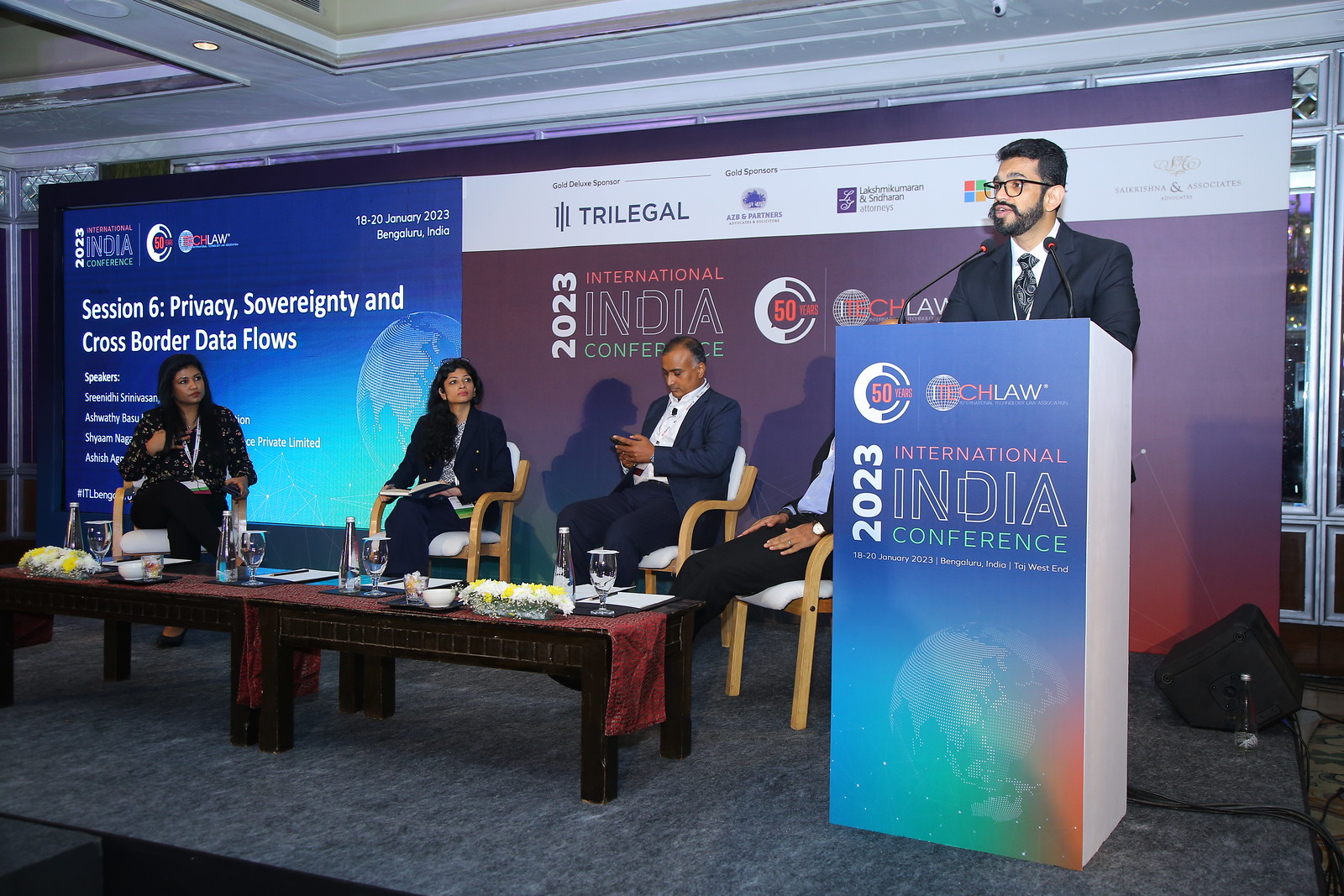The horizontally aligned rectangular image captures a scene from the 2023 International India Conference. At the forefront, a man of Indian descent is seated behind a blue podium adorned with light colors and the conference title, including "2023" vertically placed in bold white letters. He's wearing a black or navy blue suit and tie, and has short black hair, black glasses, and black facial hair including a mustache and beard. Surrounding him are four seated individuals on the right side of the stage: two men near him—one in a suit, preoccupied with his phone—and two women further left, attentively watching the speaker. The stage features a marbled dark gray and white floor, and a table covered with a dark red runner and populated with wine glasses and tea cups. Visible in the background is a large projected screen on the left, indicating "Session 6: Privacy, Sovereignty, and Cross-Border Data Flows" against a blue backdrop, while the right side reiterates "2023 International India Conference." The setting is indoors, showcasing various colors like shades of green, orange, red, and purple, as well as logos from sponsors like Microsoft and Trilegal.